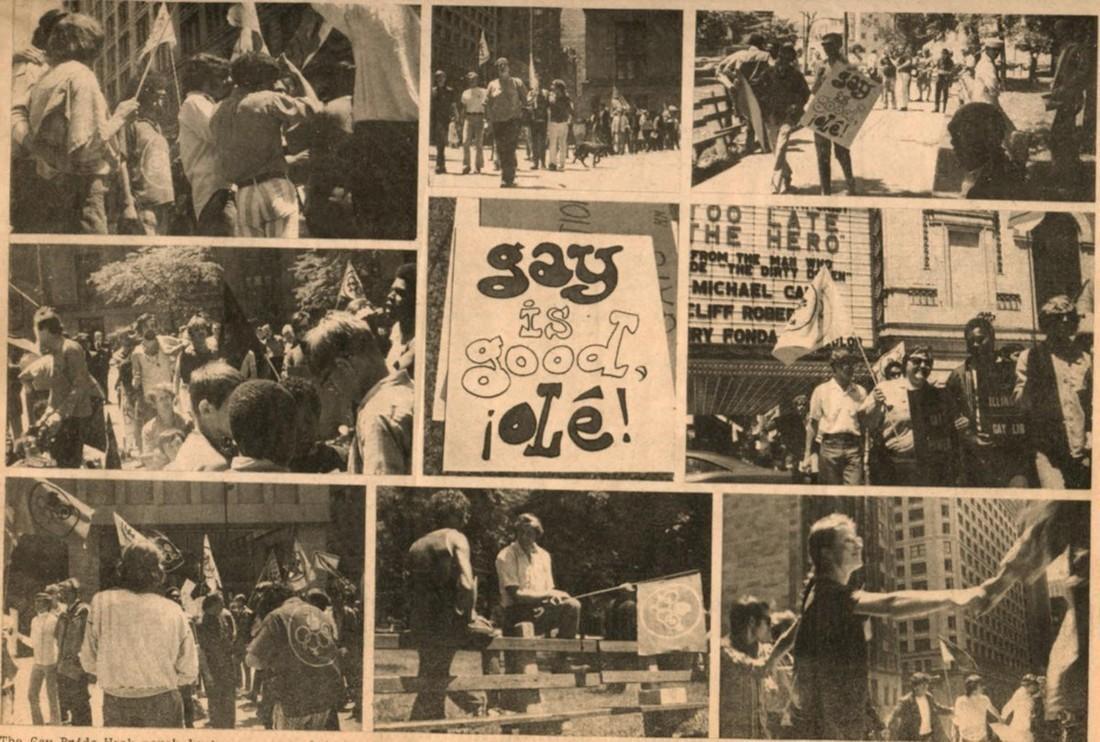This detailed poster features a collage of sepia-toned, black and white photographs depicting scenes from a gay rights rally, likely from the 1960s though some elements suggest the 1970s or 1980s. The collage contains six distinct images showing different aspects of the protest. Central to the composition is a prominent message that reads, "Gay is Good, OLE!" The poster captures a variety of scenes including individuals holding flags and banners, people walking through city streets, and protesters marching in front of a theater displaying a film titled "Too Late, the Hero." In one image, two men are seen conversing while leaning on a park bench, while another features a woman waving a flag energetically. The faded quality of the images, combined with the nostalgic sepia tone, adds to the historical and poignant nature of this vibrant and dynamic depiction of the gay rights movement.